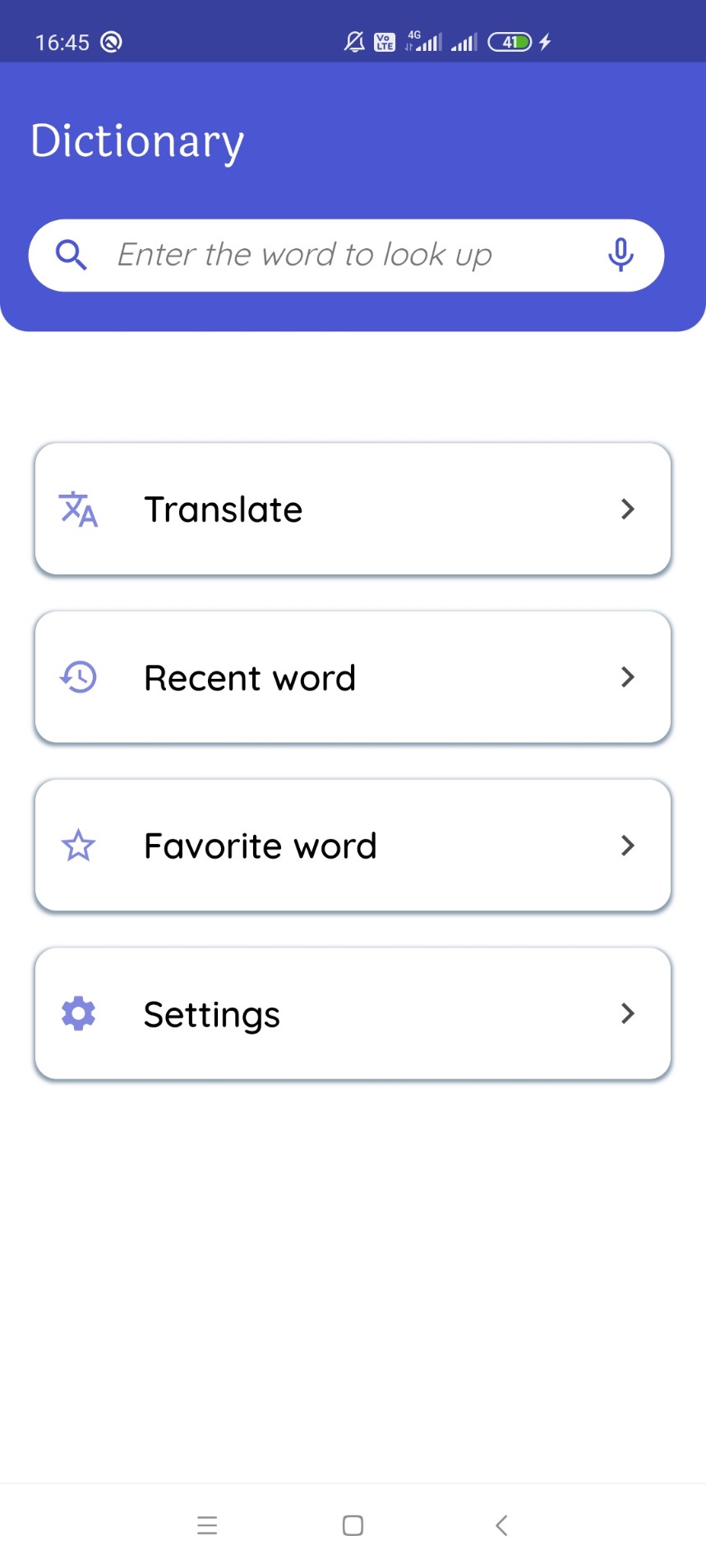This is a detailed screenshot from a person’s cell phone, displaying various interface elements and status indicators. At the top left corner, the time is shown as 16:45. Adjacent to the time is a bell icon with a slash through it, signifying that the phone is on silent mode. The phone is connected to a 4G network and has a battery level of 41%. This status information is presented on a dark blue banner.

Beneath the dark blue banner, there is a slightly lighter but still dark blue banner with the word "dictionary" written in white letters. Below this banner is a search bar prompting users to "enter the word to look up." On the left end of the search bar is a magnifying glass icon, and on the right end is a microphone icon, indicating voice search functionality.

Below the search bar are four options: "Translate," "Recent word," "Favorite word," and "Settings," each accompanied by respective icons. The "Translate" option features an icon of a Japanese character alongside the letter "A." The "Recent word" option is denoted by a clock face with a circular arrow around it, indicating history. The "Favorite word" option is marked with a star icon. Lastly, the "Settings" option is represented by a blue gear icon, signifying preferences and configuration settings.